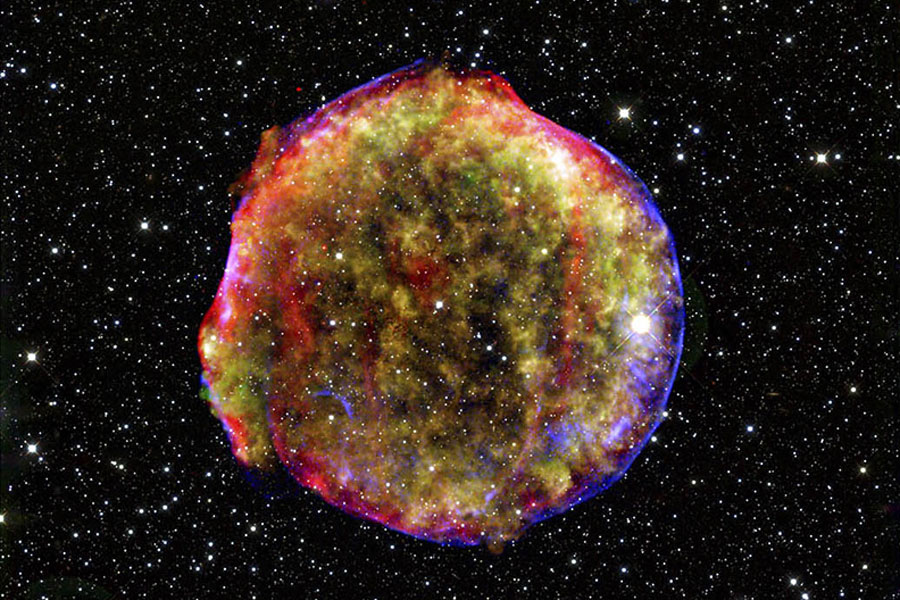This captivating image of a celestial phenomenon, likely captured via a telescope or spacecraft and digitally enhanced for vibrant detail, showcases a visually stunning scene in outer space. The backdrop is a vast expanse of deep black, studded with numerous white and blue stars, creating a sense of the infinite cosmos. 

In the center of the image lies a large, imperfectly round orb encased in a mesmerizing blue ring that shifts to violet along its edges. Inside this translucent bubble, a vivid mix of green and red gases swirl together, punctuated by a prominent yellow gaseous area. Amidst this colorful gaseous cloud, several stars are visible, with one particularly large and brilliantly bright star situated prominently to the right, emitting a glow that surpasses any of the surrounding stars. The overall effect might suggest a nebula forming, a star exploding, or perhaps an artistic interpretation of such cosmic events, merging science and imagination.